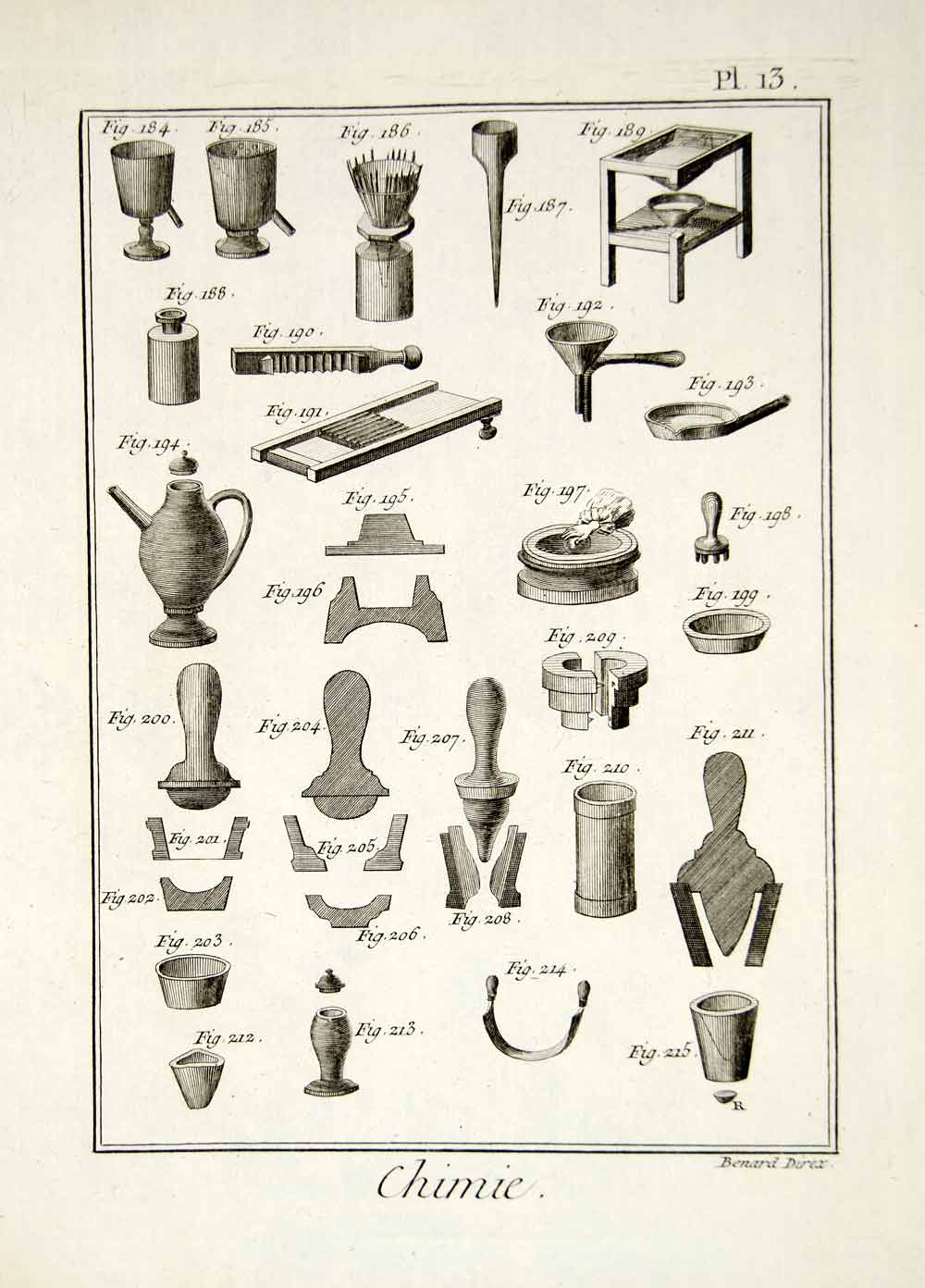This image appears to be a worn, off-white page from an old book or a tan poster showcasing the intricate works of a French metalsmith, possibly a tinsmith. The page has a delicate border surrounding an array of detailed illustrations of various metal objects, including cauldrons, vases, pots, cups, nails, screws, and clamps. Each item is meticulously labeled, albeit the labels are faint and possibly written in pencil. Prominent text includes "PL-13" at the top and "CHIMIE" written at the bottom. In the lower right-hand corner, there is a name that seems to be "Bernard Durex" or perhaps "Bernard Direx." The illustrations also feature some cross-sectional views of the objects and tools, suggesting their usage and construction within the metalwork context. The composition and style hint at historical metalworking, possibly relating to the antiquity period where a specialist like a tinsmith, known as a whitesmith, might have crafted such objects.